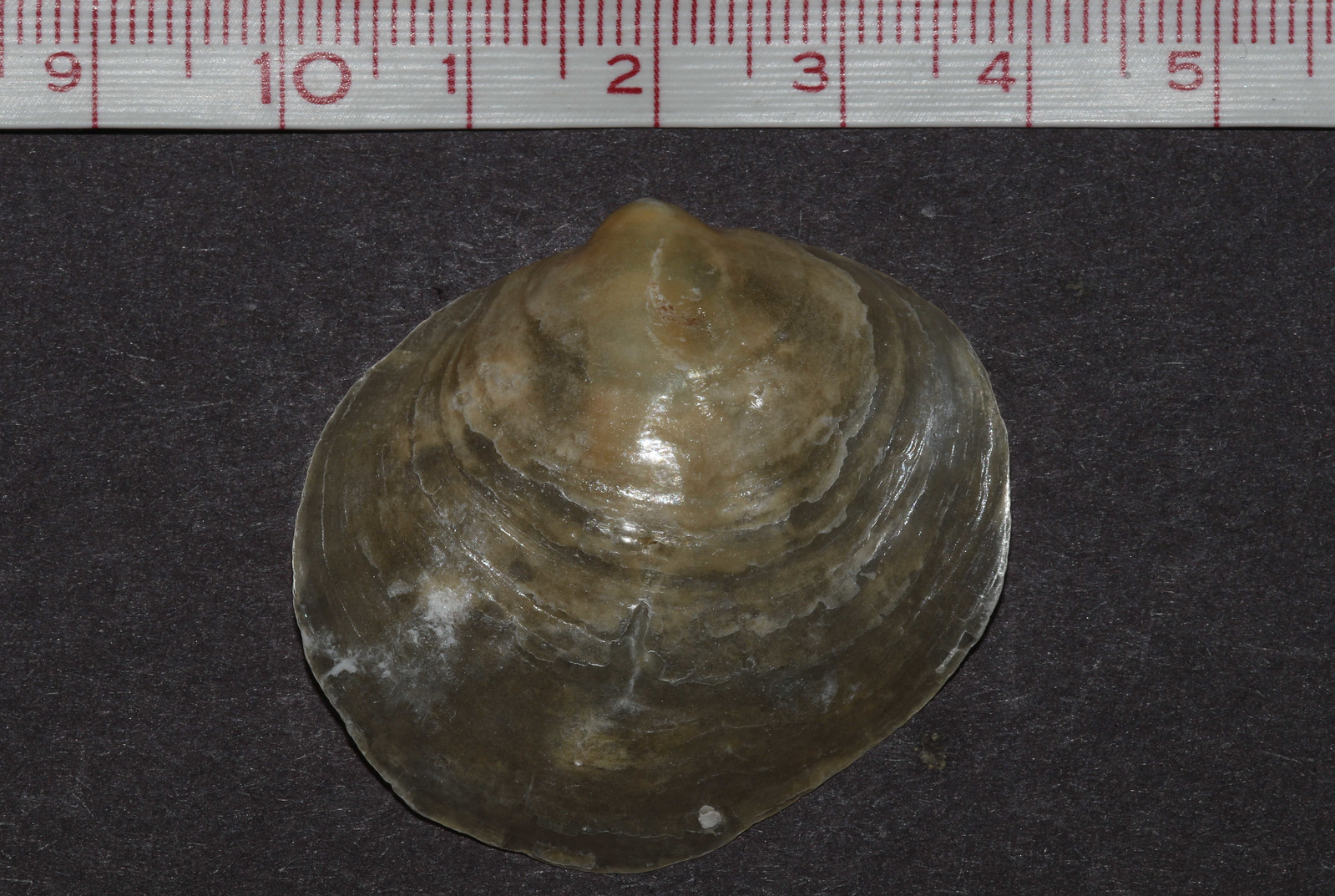This photograph features a close-up of an oyster shell, predominantly positioned at the center of the image and exhibiting various shades of brown and tan. It rests on a dark gray or off-black, slightly textured surface. Above the oyster shell lies a white fabric ruler marked with crimson-colored centimeter and millimeter notations, suggesting an attempt to measure the shell's size. The absence of any visible text in the image and the meticulous arrangement of the objects indicate that the setting may be indoors, possibly within a scientific context. The overall color palette of the image includes shades of red, white, black, brown, and tan.